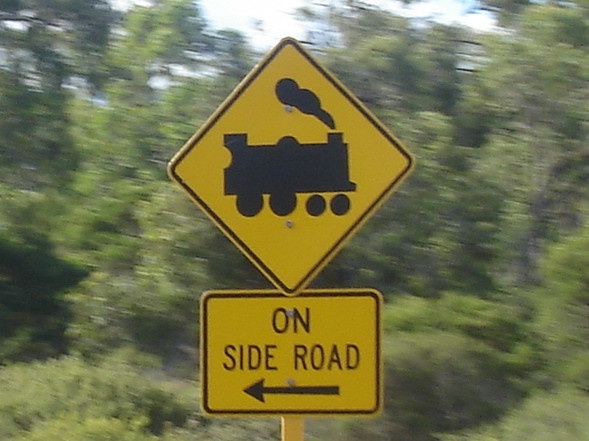A public traffic sign is prominently displayed against a backdrop of lush greenery, including trees, bushes, and grass basking in the daylight under a clear sky. The sign itself is set in a diamond shape with a vivid yellow background. At the center of this diamond, there's a black silhouette of a train car emitting a small plume of smoke. A thin black stripe outlines the edge of the diamond, adding to the sign's visibility. Directly beneath this train symbol, another yellow sign with a similar black border sits. This sign bears the words "ON SIDE ROAD" in bold black letters and features a left-pointing arrow, indicating the direction of the side road where the train operates.